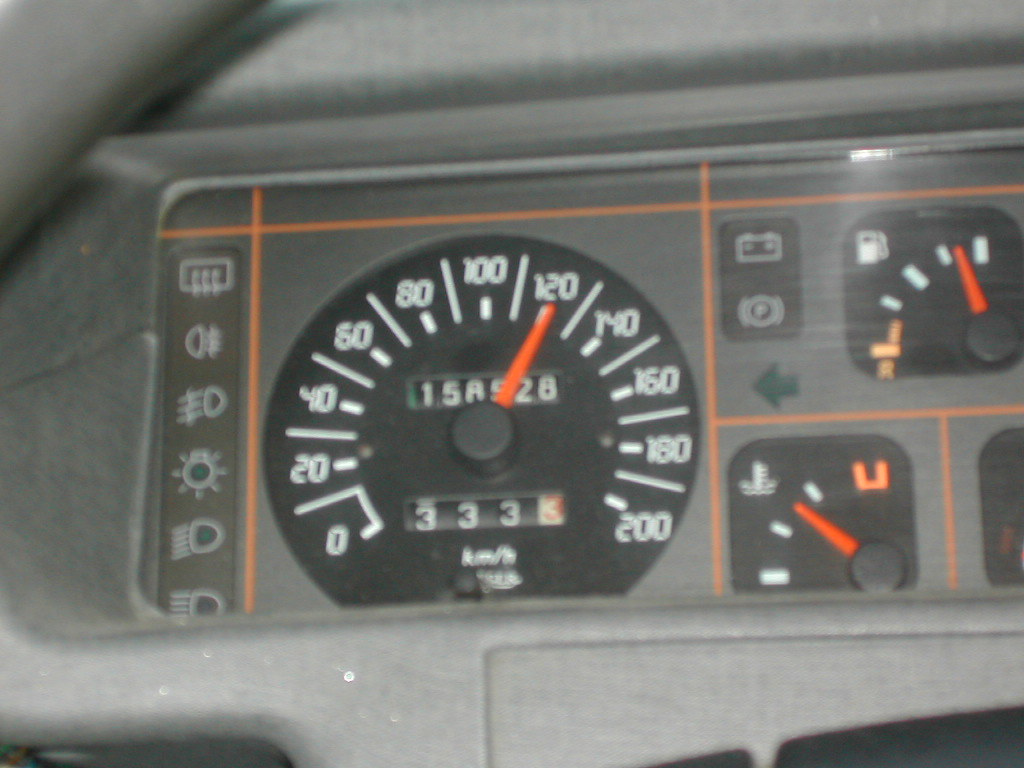A detailed view of a car's dashboard within a gray interior. The dashboard features a rectangular display area, segmented by a thin orange line, housing multiple gauges and indicators. On the left, several icons represent various functions: headlights, high beams, and a lamp. Adjacent to these icons is the speedometer, calibrated in kilometers per hour and ranging from 0 to 200. Centrally positioned within the speedometer is the odometer, displaying a total distance of 158,528 kilometers traveled. To the right of the speedometer, indicators for the battery and parking brake can be seen. Further right is the fuel gauge, showing approximately three-quarters full, and below it, the oil gauge, indicating a level at about halfway up.